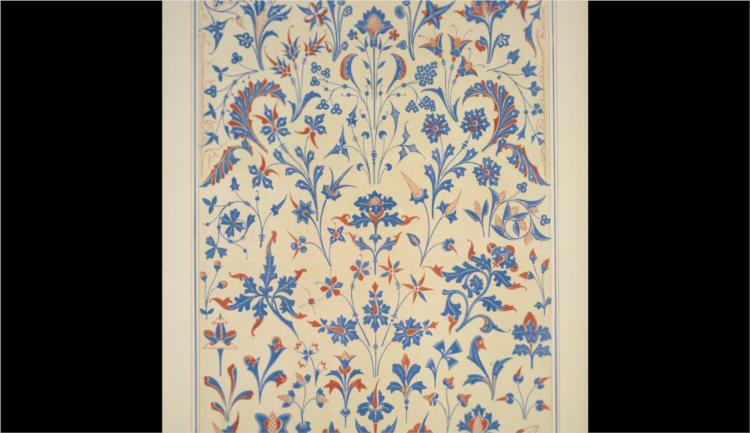This image features a highly detailed artwork bordered by black bars on both sides. The central section presents a striking contrast with a clean white base, framed by a fine blue line and a cream-colored background. The artwork itself resembles a meticulously crafted piece that could serve as wallpaper, art, or even a book cover. It showcases an array of intricately drawn flowers and leafy patterns in shades of blue, rust, and gold. The flowers, while not representing specific real-life species, exhibit a variety of forms and styles, from feather-like plants to shapes resembling irises and daisies, with some petals featuring a pink tint. The detailed designs are repeated across the canvas, showing a mix of geometric shapes and natural forms that create a harmonious yet complex visual tapestry.